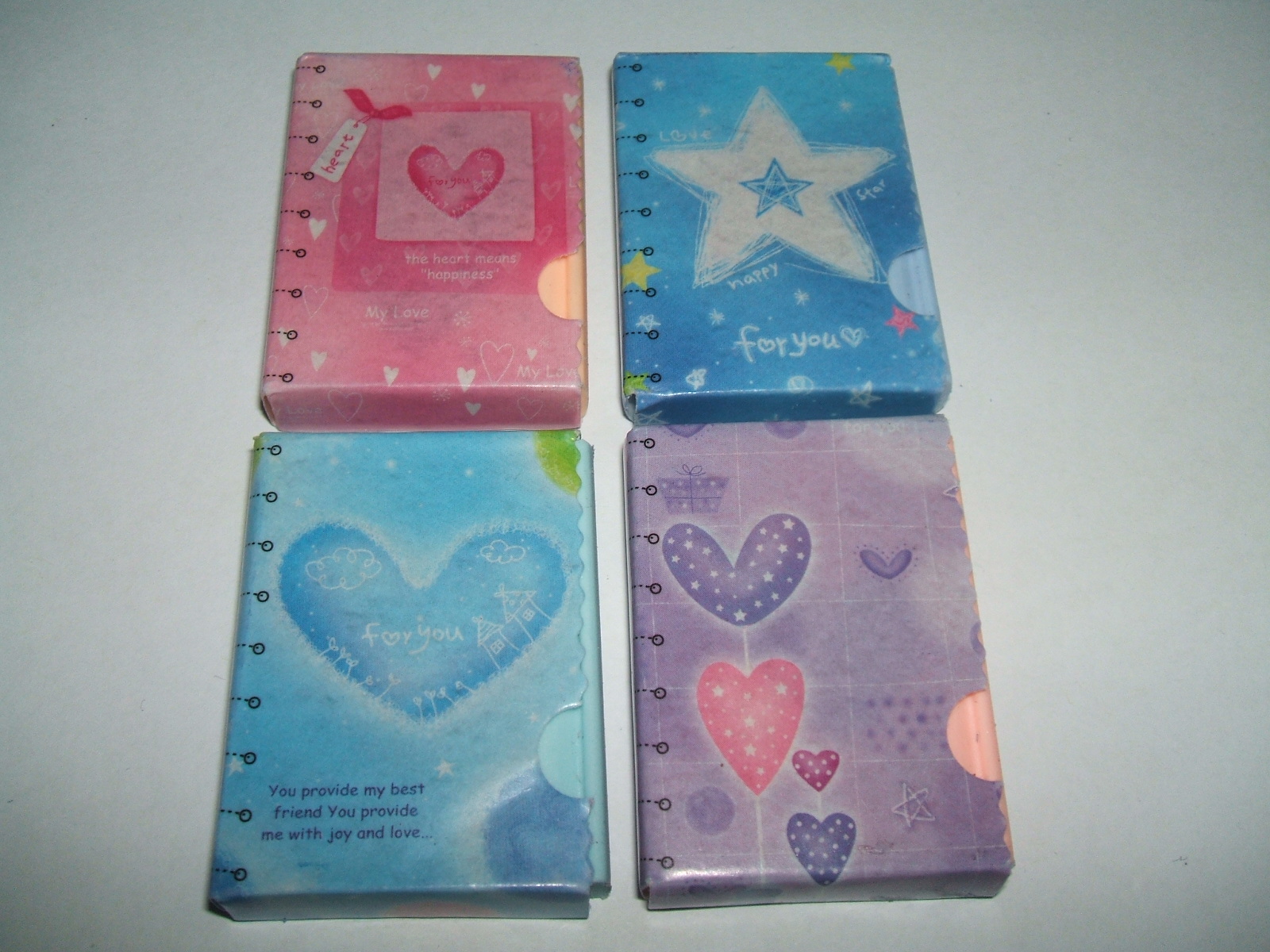The image displays four small, colorful notebooks arranged in a square formation on a white surface, each featuring distinct wrapping paper designs. The top-left notebook is pink and decorated with metal spirals, hearts, and the phrases "The heart means happiness" and "My love" written repeatedly alongside various heart patterns. The top-right notebook, dark blue in color, showcases a star with a smaller star inside, accompanied by the words "Love star happy" and "For you." The bottom-left notebook is light blue, adorned with a prominent heart and the inscription "You provide my best friend, you provide me with joy and love." Finally, the bottom-right notebook is purple, featuring pink and purple hearts, some of which have stars inside them. These diaries, designed with a child-like aesthetic, combine to create a vivid and sentimental tableau.